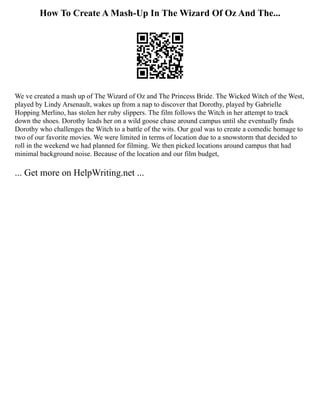The image features a central, black-and-white QR code with no border, set against a white background. Above the QR code is a title in normal black font that reads, "How to Create a Mash-up in the Wizard of Oz and the..." Centered underneath the QR code, there's a left-aligned paragraph detailing the project: "We've created a mash-up of the Wizard of Oz and the Princess Bride. The Wicked Witch of the West, played by Lindy Arsenault, wakes up from a nap to discover that Dorothy, played by Gabriel Coppine-Merlino, has stolen her ruby slippers. The film follows the witch in her attempt to track down the shoes. Dorothy leads her on a wild goose chase around campus until she eventually finds Dorothy, who challenges the witch to a battle of wits. Our goal was to create a comedic homage to two of our favorite movies. We were limited in terms of location due to a snowstorm that rolled in the weekend we had planned for filming. We picked locations around campus that had minimal background noise due to our film budget." At the bottom left corner of the image, the text reads, "Get more on helpwriting.net," in a slightly larger font than the rest of the paragraph.